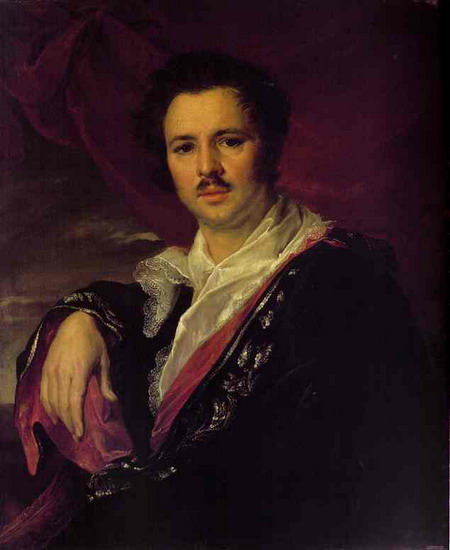The painting depicts a middle-aged, upper-class man with short, dark hair and a small mustache with a unique gap in the middle. His dark eyes and slightly sad expression are directed at the viewer, creating an engaging and contemplative atmosphere. He is dressed in a luxurious, dark, flowing robe that reveals a red inner lining, paired with a white, silk-looking undershirt featuring a lace collar. His right arm is draped over what appears to be an armrest, with his hand hanging down in a relaxed manner. The background is a mix of indistinct, flowy elements, possibly representing a sky with dark purple and gray clouds or rich, flowing curtains, adding an air of mystery and depth to the scene. The overall composition and his regal attire suggest he is an aristocrat, portrayed with intricate detail and emotional depth.